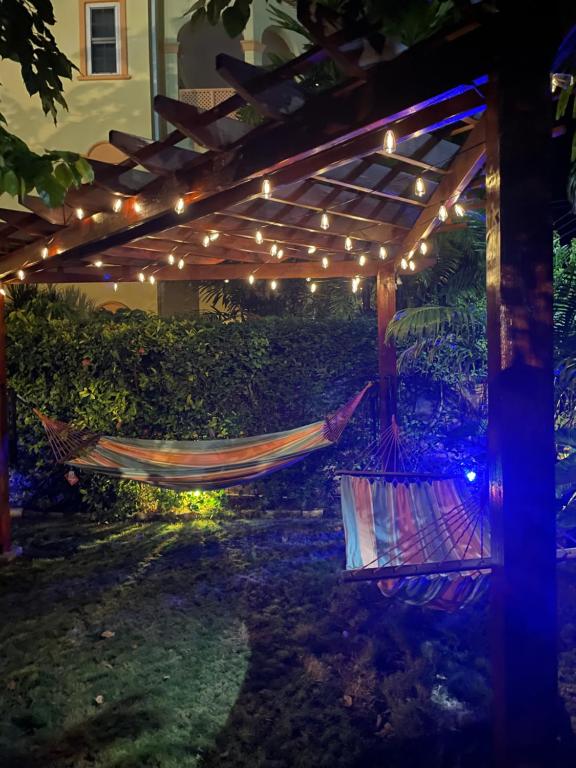The image captures a nighttime scene of an inviting outdoor patio featuring a wooden cabana with a triangular roof. Two colorful, canvassed hammocks, decorated in a vibrant pattern of blue, yellow, green, orange, red, and purple, hang perpendicularly from sturdy vertical and horizontal wooden beams. Fairy lights dangle gracefully from the structure, casting a warm glow on the surroundings. The cabana is nestled amidst lush greenery, with many plants encircling the cozy setup. In the background, a yellow building reminiscent of a hotel, complete with yellow windows and a second-floor balcony, peeks through a dense wall of trees. This serene setting exudes a relaxing and enchanting atmosphere.